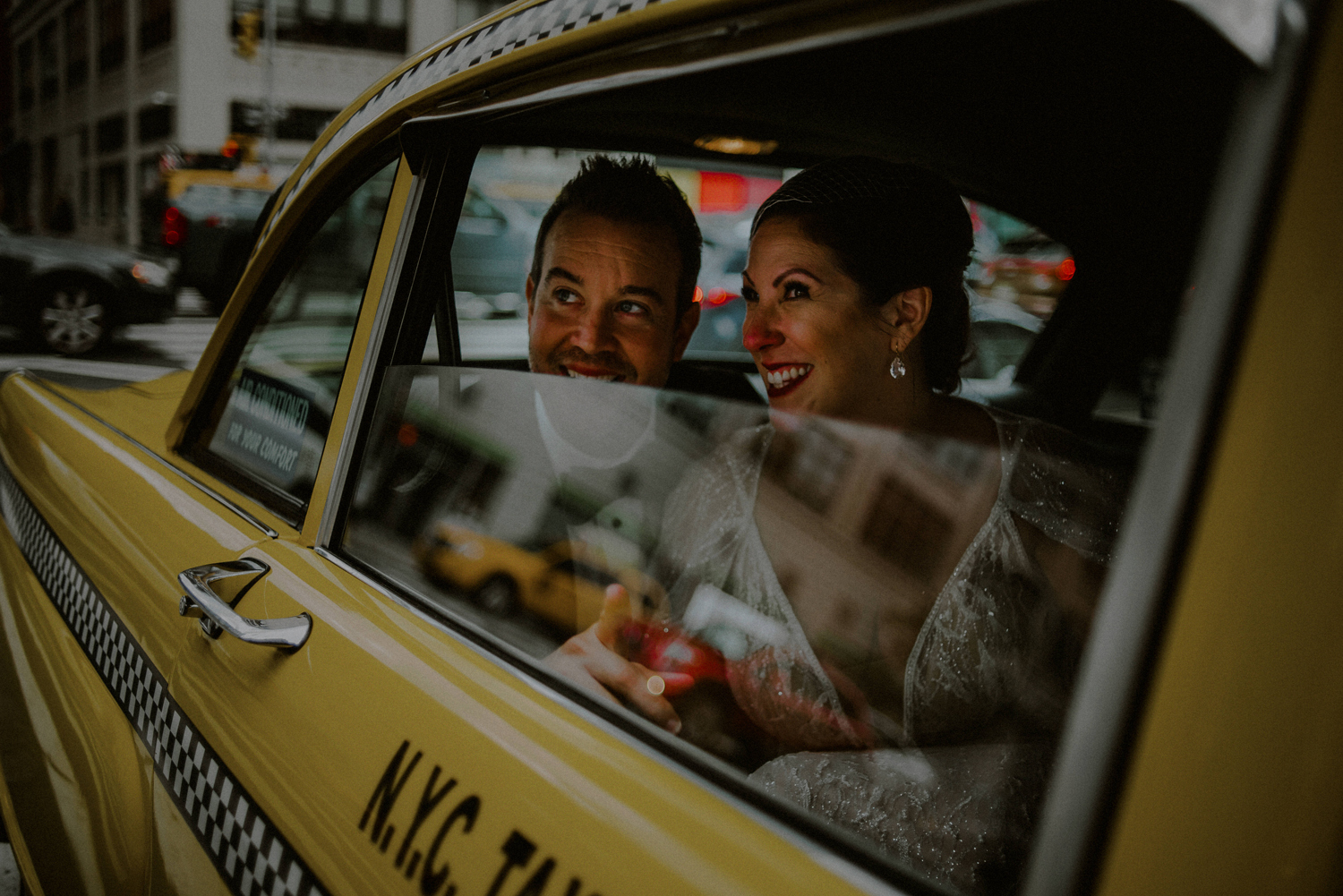This vibrant color photograph captures a newlywed couple in the back of a classic 1950s style New York City taxi. The iconic yellow cab, bearing the distinctive NYC logo and a black-and-white checkered stripe, has its window rolled halfway down. Inside, the groom sits on the left, characterized by his dark short hair, wrinkled forehead, and dressed in a black suit jacket, black bow tie, and white dress shirt. The bride, seated to the right, sports an elegant updo and sparkling earrings, and is adorned in a v-necked wedding gown with silver and white details. Both are smiling broadly, exuding joy as they hold hands and look out the window at the bustling city street, where blurred cars indicate the lively background. The intimate close-up further accentuates the couple's happiness and the celebratory atmosphere of their special day.